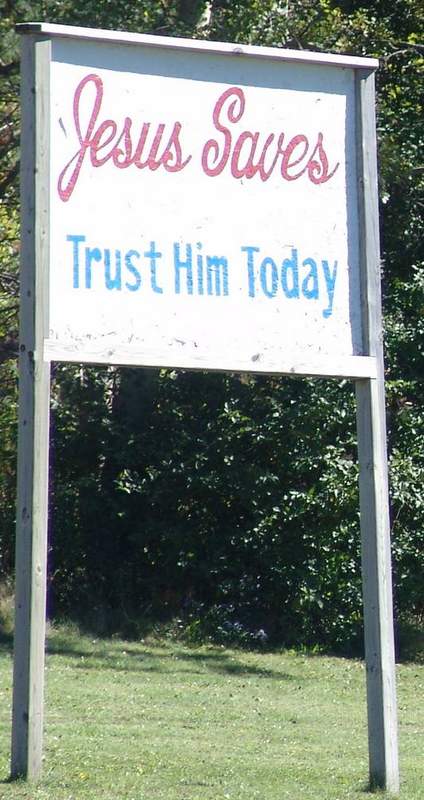The image showcases an outdoor sign prominently displayed in a sunny setting. The sign is supported by two sturdy wooden two-by-fours that are firmly embedded into the ground. The sign itself is suspended between these two posts and is further stabilized by an additional horizontal wooden piece at the top. In elegant red cursive letters, the sign reads, "Jesus Saves." Below this, in bold blue block letters, it states, "Trust Him Today."

The photograph captures the bright daylight with the sun casting clear, well-defined shadows of the sign onto the ground. The sign is positioned amidst a patch of well-maintained, neatly trimmed grass, adding to the overall serene and orderly appearance. The background is lush with greenery, featuring an array of bushes and trees adorned with vibrant green leaves, contributing to the natural and tranquil outdoor setting.